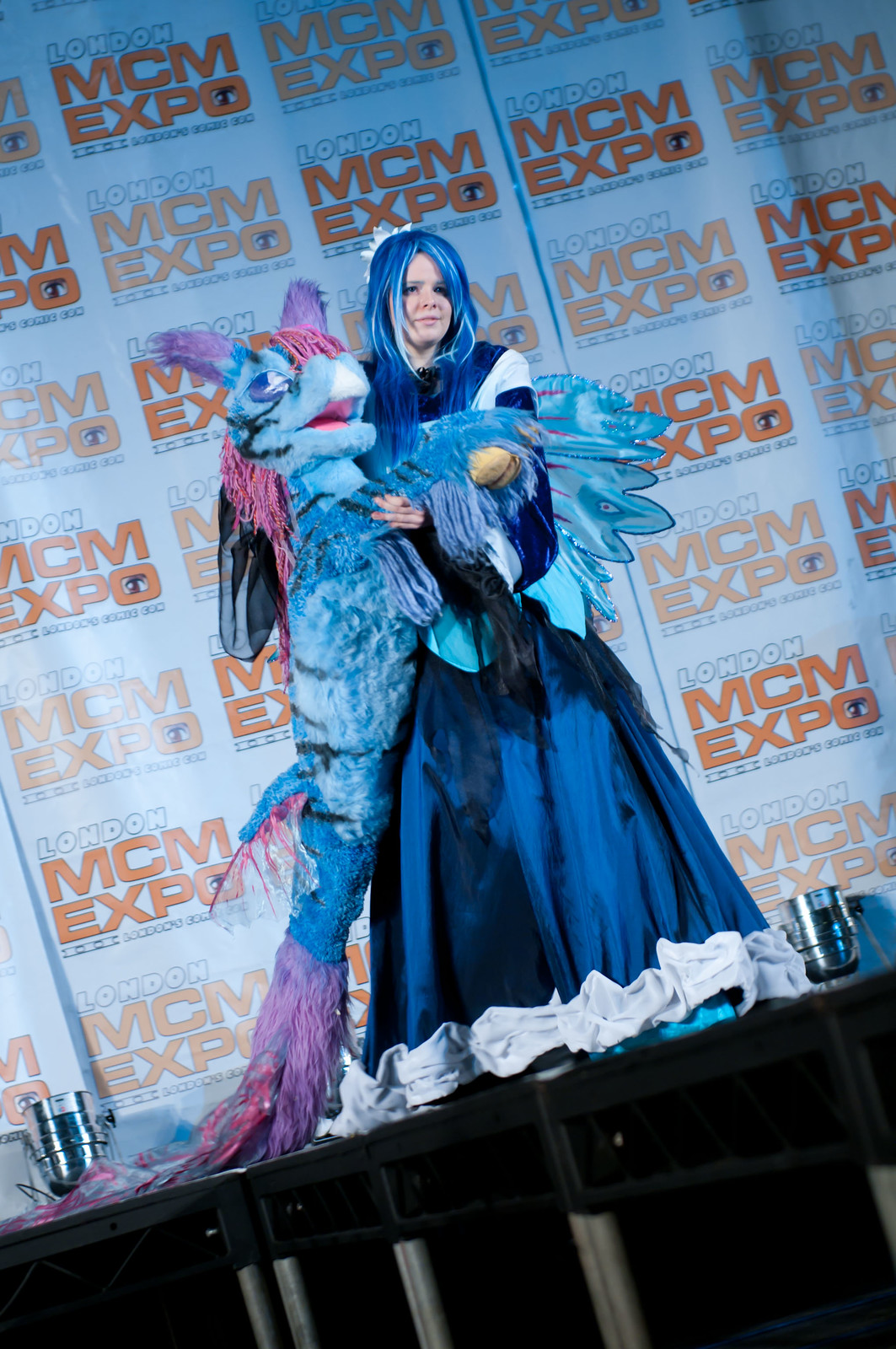The photograph captures a vibrant scene at what appears to be the London MCM Expo, likely taken during some form of character or anime convention. Central to the image is a woman standing on a black stage, beneath which metal supports are visible. She is dressed in a long, elegant blue gown, her ensemble augmented with a blue wig and a white flower tucked into her hair. Intriguingly, she also sports large blue wings extending from her back.

She is holding a distinctive blue plush horse, which is anthropomorphized and has black stripes, purple hair, and violet fur along its hind legs. This stuffed creature has its blue hooves in her arms as they pose together. The horse's ears and tail are of different shades of purple and pink, adding to its colorful appearance. 

Behind them, the backdrop is a white display repeatedly adorned with the text "London MCM Expo" in orange and white letters, and "London's Comic Con" also appears prominently. Bright stage lights are seen on either side, highlighting the duo as they take the central focus of this lively convention setting.